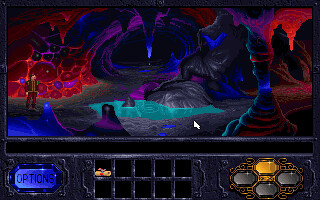A pixelated video game scene featuring a vibrant, multi-colored cave system. The cave walls are a mix of red, purple, and blue hues with a bubbly texture. Sharp spikes hang menacingly from the ceiling and jut out from the ground, adding an element of danger. At the center of the scene, a blue puddle of water contains a single gray spike emerging from it.

To the left, a character stands dressed in red pants and a red jacket with gold trim, complemented by a green undershirt. The character has short brown hair. The interface displays "Options" in black text on a blue gem in the bottom left corner. To the right of the screen, there are ten black squares; the top left square contains a scroll tied with a red ribbon. In the bottom right corner, four gems are displayed, three of which are gray, while the top gem is gold, all adorned with gold trim. A white pointer is positioned in the middle of the screen, likely controlled by the player.